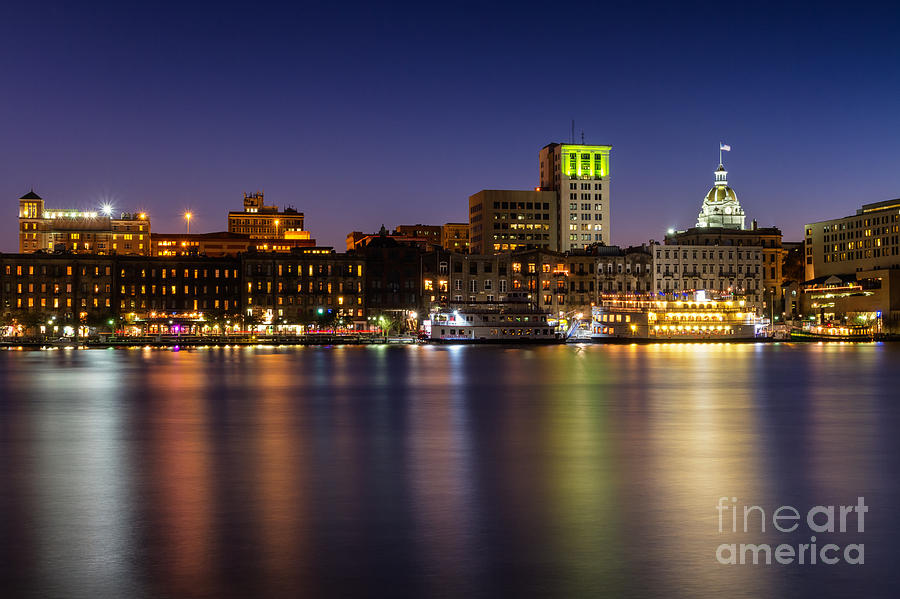This nighttime outdoor image showcases a beautifully illuminated cityscape centered above a calm body of water, reflecting the vibrant lights of the buildings. One standout structure features a dome-shaped top, while another has a striking bright green-lit pinnacle. A dock with boats is visible in the distance, adding to the serene aquatic setting. The scene is accentuated by a range of colors including blue, green, gray, white, yellow, pink, purple, and tan, creating an artistic and captivating visual. "Fine Art America" is prominently watermarked in the bottom right corner, indicating the image is likely from a poster or print.